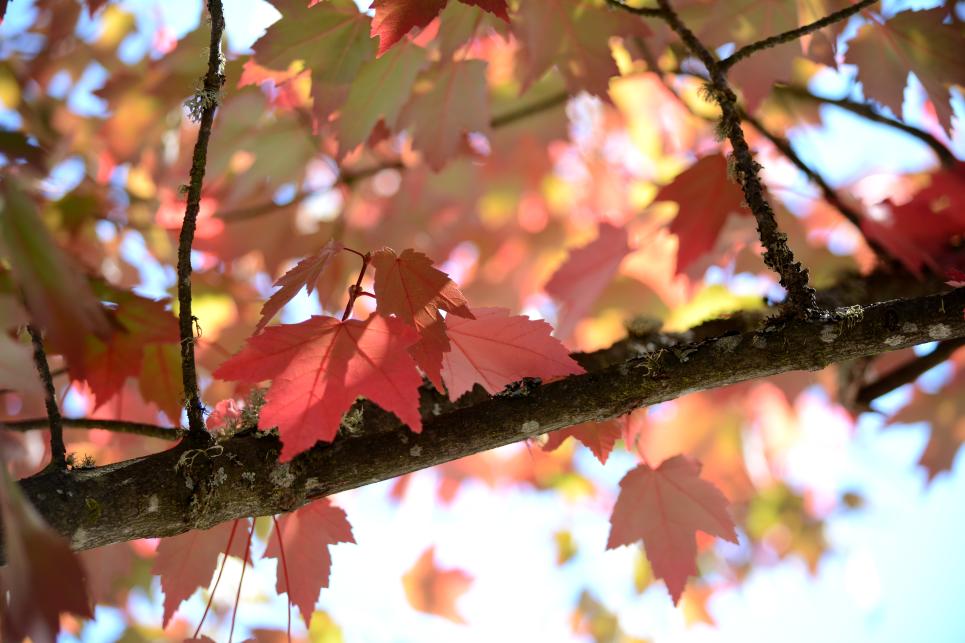This photograph captures the serenity of nature in autumn. The angle looks upward through the lower branches of a tree, showcasing a vivid tapestry of red and yellow leaves that signal the changing season. The contrasting blue sky above is dotted with soft, white clouds, adding depth to the scene. A brilliant white light pierces through the foliage at the bottom of the image, creating a striking interplay of light and shadow. The main branch, a mix of brown and gray hues, stretches horizontally across the frame and sprouts into thinner twigs that rise upwards, each adorned with clusters of leaves. The red leaves dominate the foreground, while patches of yellow peek through in the background, highlighting the tree's natural gradient. This intricate composition celebrates the beauty of autumn in splendid detail.